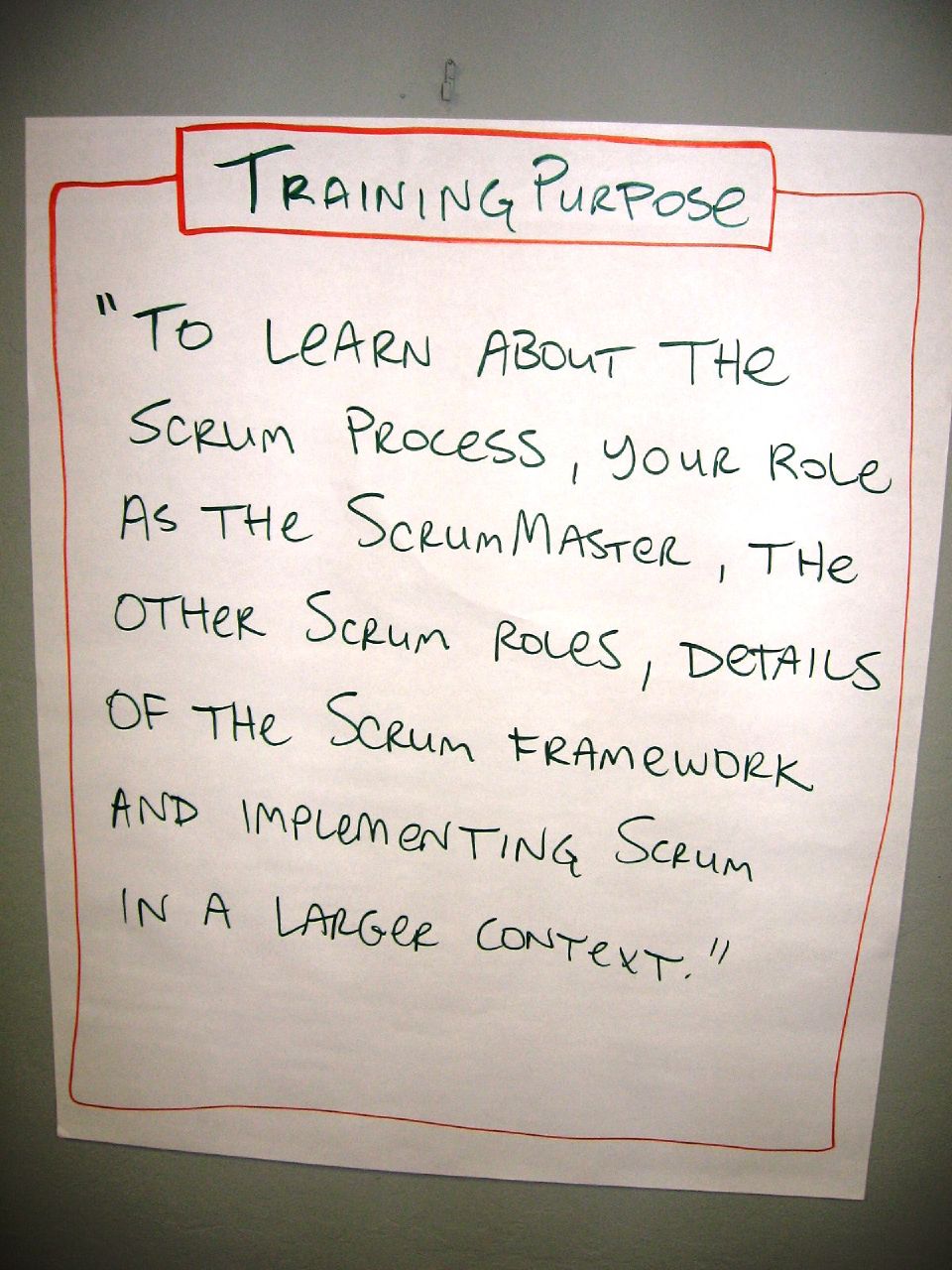The image displays a white piece of paper affixed vertically to a gray wall, likely for instructional purposes. The paper is surrounded by a hand-drawn orange border that runs along its edges. At the top of the paper is a thicker, red rectangular box containing green, freehand text that reads "Training Purpose." Below this, additional green, handwritten text is spread out across the page, enclosed within the orange border. The text reads: "To learn about the Scrum process, your role as the Scrum Master, the other Scrum roles, details of the Scrum framework, and implementing Scrum in a larger context." Notably, all the text appears to be written in green marker. Above the top of the paper, there is a small indent in the wall, indicative of a minor repair. Shadows are discernible in the corners of the paper, especially towards the bottom.